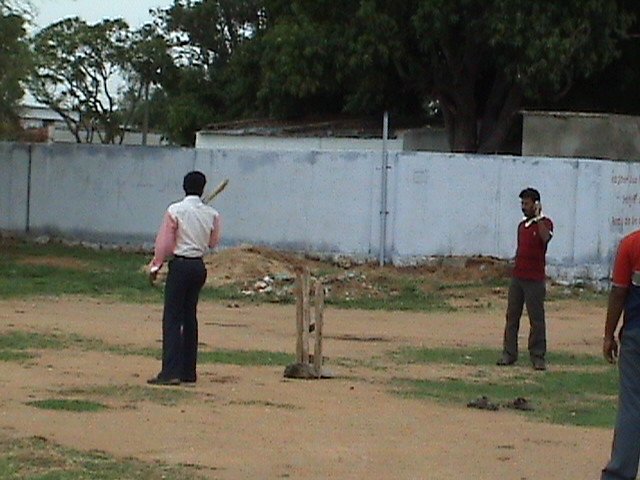This is a detailed full-color photograph captured outdoors during the day, depicting a cricket match on a primarily dirt field with sparse patches of grass. The scene includes three men: on the left, a man with short dark hair, wearing black pants and a white shirt with pink sleeves, is holding a cricket bat in front of the wooden cricket stumps. To his right, another man with a dark complexion, possibly Indian, is wearing a purple shirt with a white collar and brown pants and is holding a phone to his ear. The third man on the far right, partially captured in the frame, has brown hair and is wearing a red shirt and blue pants. In the background, a large gray cement wall with red markings stretches across, with green leafy trees and the tops of white-roofed buildings visible behind it. A small wooden structure, possibly part of the cricket setup, stands between the first two men. The sky in the upper left corner of the image is a clear blue, contrasting with the earthy tones of the playing field. Casual footwear, possibly sandals, are scattered in the vicinity, adding to the informal and relaxed setting, hinting at a leisurely game of cricket.